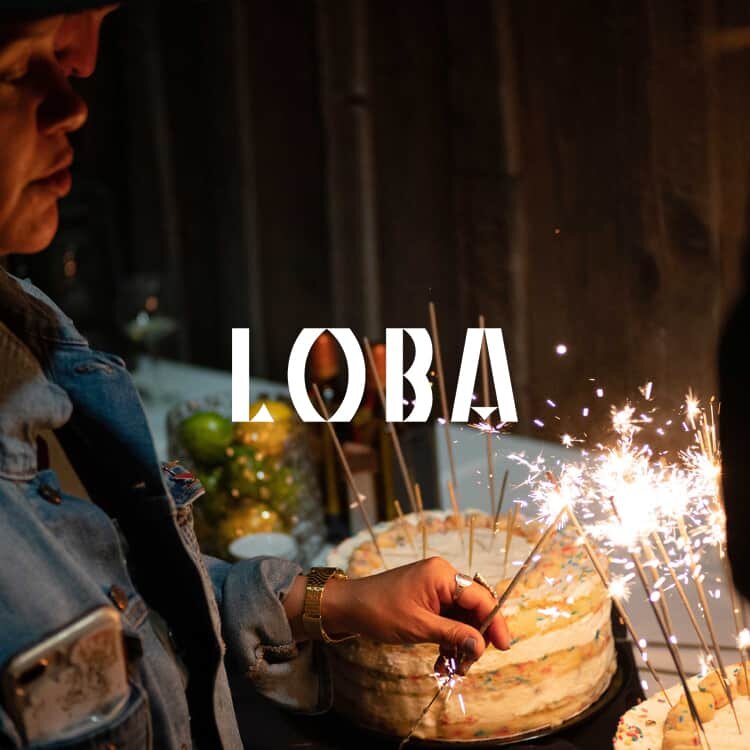The image captures a vibrant celebration scene, likely a party or birthday event, with a festive atmosphere suggested by the numerous sparklers. Central to the composition is a woman positioned on the left, dressed in a jean jacket with a cell phone tucked in her front pocket. She's engaged in lighting sparklers, one of which she holds in her hand. Notably, she wears a wristwatch and a ring, adding to her casual yet festive ensemble. 

On the table before her, adorned with a white tablecloth, sit two cakes. The cake in the foreground is sprinkled with unlit sparklers, featuring light, pink, and orange accents, while the cake slightly to the right is aglow with sparklers, emitting bright, white sparkles. A container of fruit also rests on the table, providing a touch of color and variety. 

In the backdrop, wooden panels add a rustic charm to the setting. Dominating the center of the image, in a bold and angular white font, the word "LOBA" (L-O-B-A) is prominently displayed, possibly hinting at a theme or name associated with the event. The photograph, taken at night, employs a realistic, representational style, capturing the essence of the moment in vivid detail.